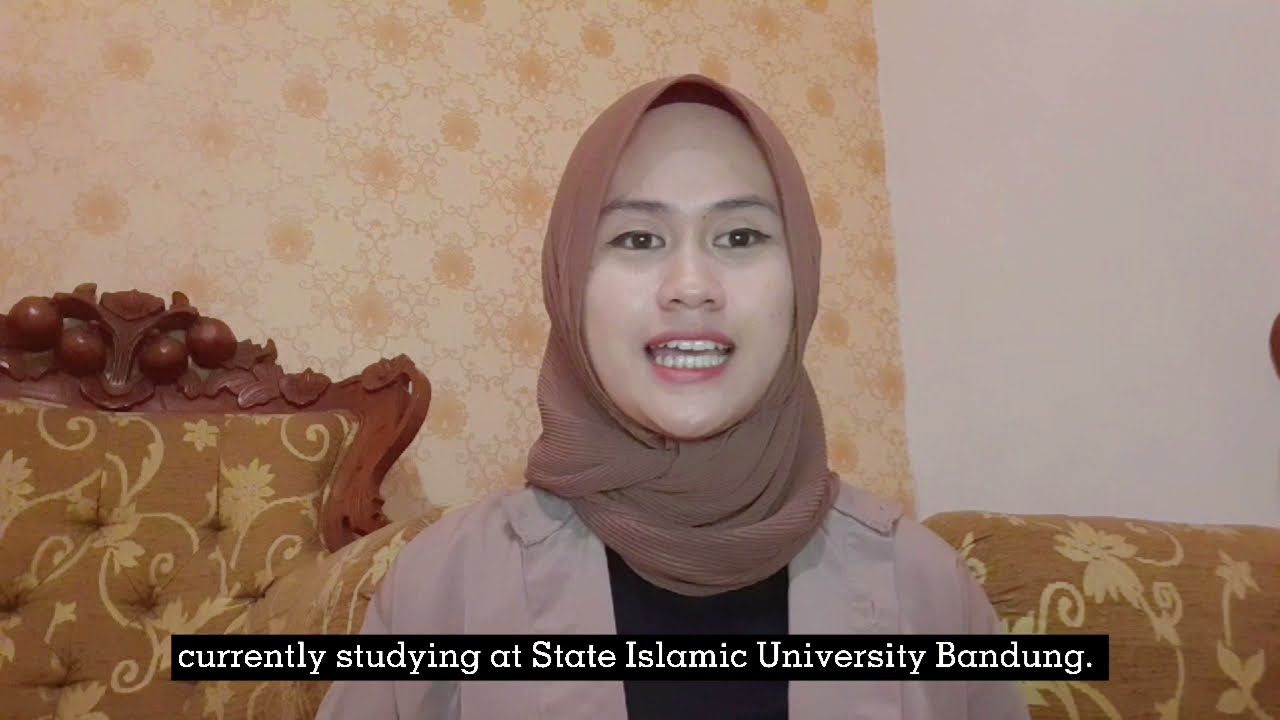In the image, a woman is seated on an ornate brown couch adorned with subtle floral designs. She's wearing a large headscarf in shades of purple and a light tan or rose-colored jacket over a black shirt. She appears to be speaking, her mouth open and teeth visible, likely captured during an interview. A small black rectangle with white text at the bottom of the image states, "currently studying at State Islamic University, Bandung." Behind her, the setting includes a cream-colored wall and another wall with a geometric-patterned wallpaper in shades of tan and peach. To her left, there’s another matching chair with a wooden frame featuring carvings of fruit and leaves, and both pieces of furniture share the same floral upholstery design. The scene has a warm, homely ambiance, enriched by the intricate patterns and detailed decor.